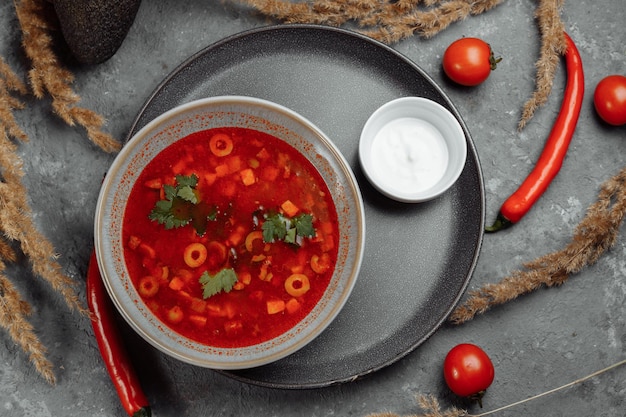In this image, we have a detailed presentation of a tomato-based soup, prominently displayed in a large, white-grayish bowl with a tan rim. The bowl is filled to the brim with vibrant red tomato juice, diced tomatoes, cilantro, and possibly some olives, garnished with chopped green herbs. The bowl is set on a black serving tray. Adjacent to the main dish, there is a smaller white bowl containing a thick white substance, potentially sour cream or another type of sauce. 

The scene is further enriched by its stone or cement background, which features scattered, uncut fresh tomatoes and long red peppers, hinting at the ingredients used in the soup. Additionally, pieces of wheat and some brown plants are placed on the left and right sides of the table, adding a rustic touch to the setting. The entire composition suggests a hearty, traditional tomato soup, emphasizing its fresh ingredients through the surrounding produce.